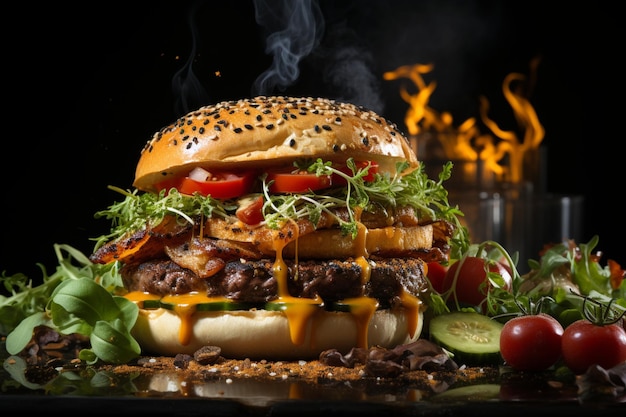The image showcases an extremely appetizing, loaded cheeseburger set against the dramatic backdrop of a blazing fire, likely from a fire pit, with vivid orange and yellow flames. Dominating the foreground, the cheeseburger boasts a glossy brioche bun generously sprinkled with black and white sesame seeds. The burger is a masterpiece, featuring thick, juicy meat patties layered between fresh, crisp tomatoes, vibrant mixed greens, cucumbers, and possibly thyme or bean sprouts. A rich, yellow cheese or mustard sauce oozes enticingly from the burger, adding to its allure. Surrounding the burger, a variety of fresh vegetables are arranged on the table, adding a touch of color and freshness to the scene. The entire setup, complete with the dripping sauce and toasted bun, lends to the impression of a high-quality, mouth-watering burger reminiscent of a gourmet restaurant offering.